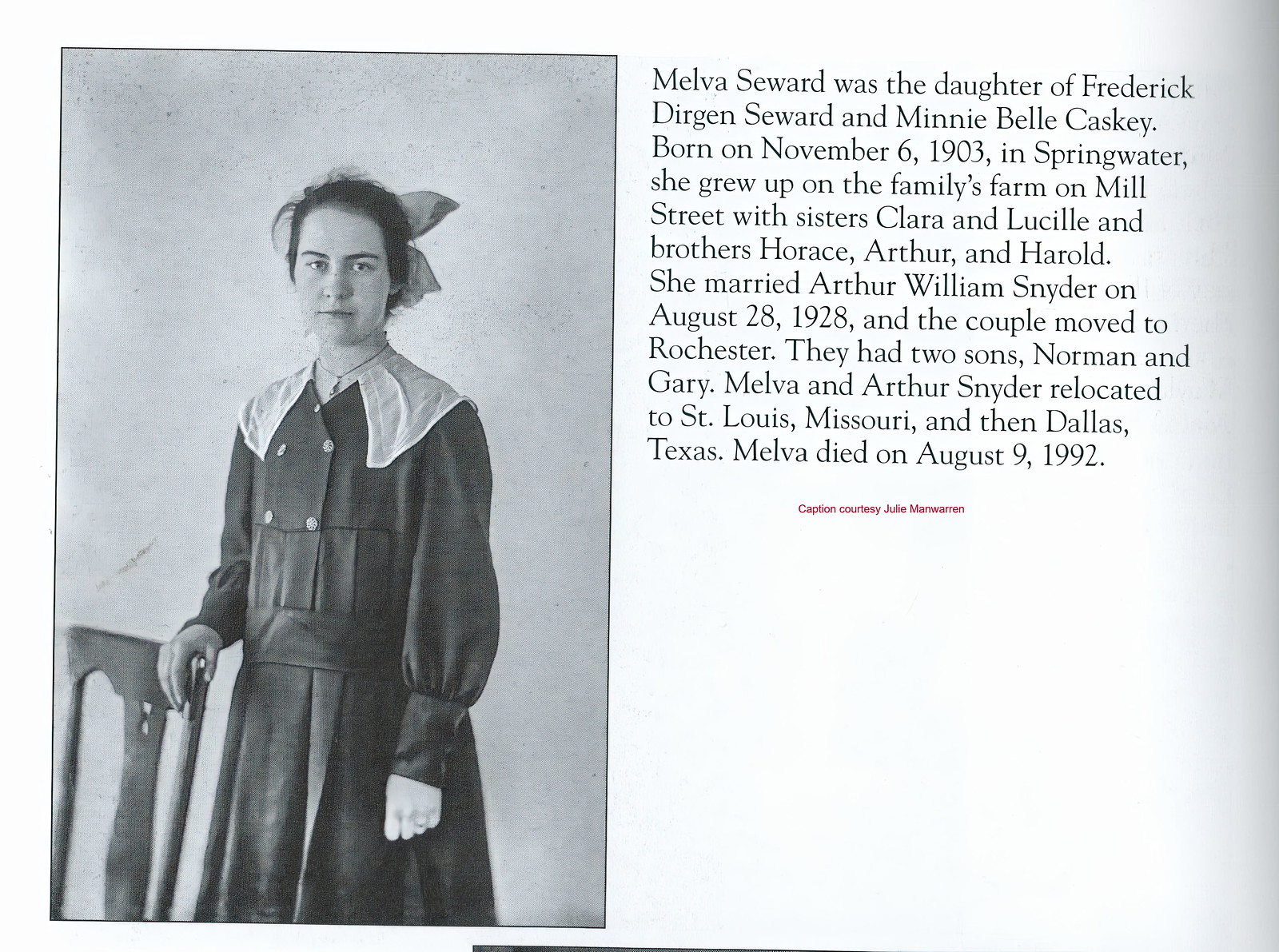The image, appearing to be a very old black-and-white photograph, features a young girl, Melva Seward, standing on the left-hand side. She is dressed in an old-fashioned, long-sleeved dark dress adorned with a white collar and has her hair pulled back with a bow. Her right hand rests on a wooden chair as she gazes neutrally at the camera. To the right of the photograph, an extensive biographical caption details Melva's life: she was born on November 6, 1903, in Springwater to Frederick Durgin Seward and Minnie Bell Caskey. She grew up on the family farm on Mill Street alongside her sisters Clara and Lucille and brothers Horace, Arthur, and Harold. Melva married Arthur William Snyder on August 28, 1928, and the couple moved to Rochester, where they had two sons, Norman and Gary. The family later relocated to St. Louis, Missouri, and then Dallas, Texas. Melva passed away on August 9, 1992. The caption credits Julia Maron for its provision.